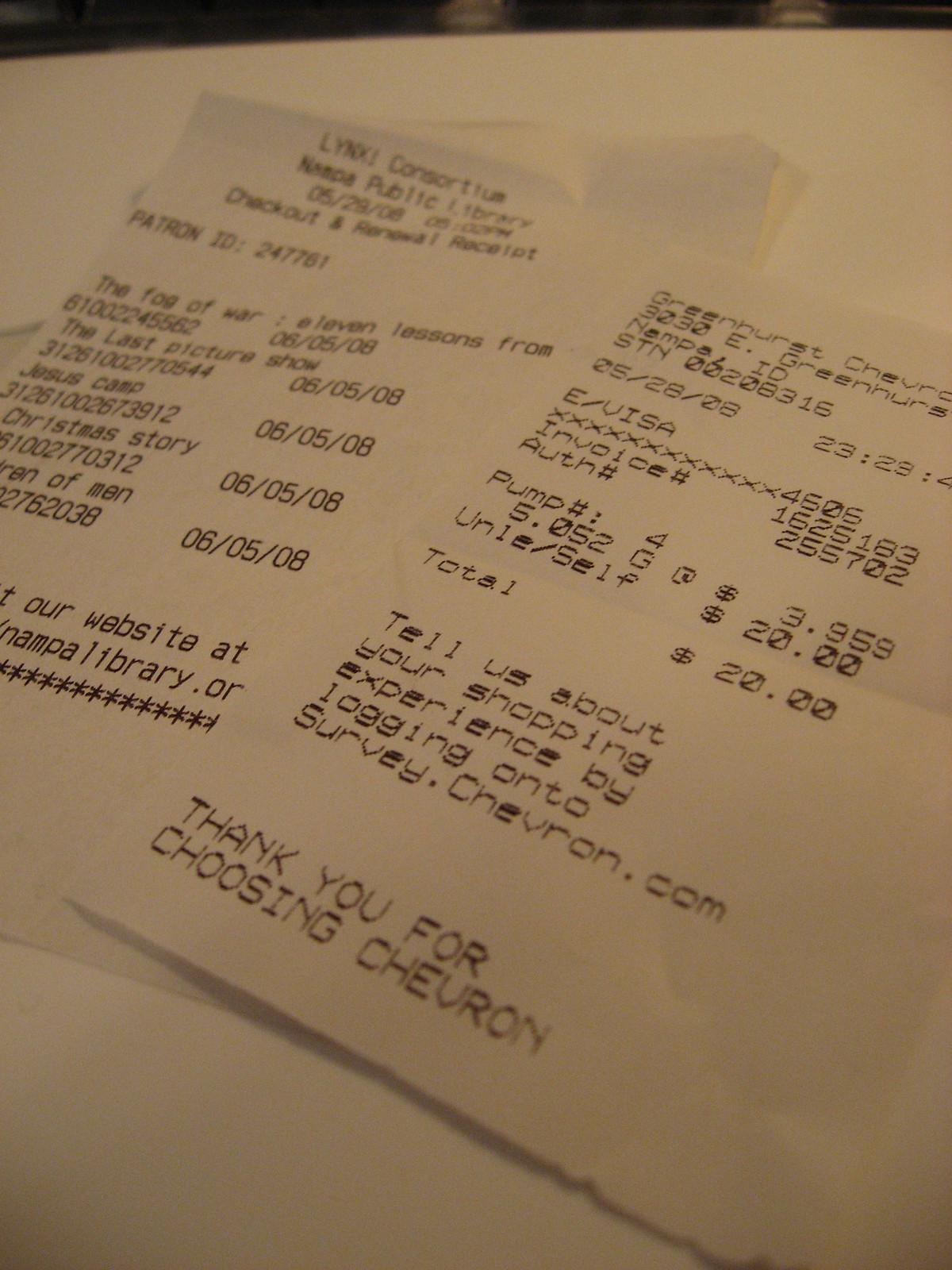In this close-up photograph, we see two receipts on a white surface, presumably a table. The receipt on the left, partially obscured by the one on the right, is from "Lynxi Consortium Nampa Public Library" dated 05/29/08. It lists several checked-out books including "The Fog of War: 11 Lessons", "The Last Picture Show", "Jesus Camp", and a partial title that might be "Siren/Men". Each book is accompanied by a unique identification number and the due date of 06/05/08. The receipt also includes a patron ID and partially visible website link to nampalibrary.org.

The second receipt on the right is from "Greenhurst Chevron", a gas station where the patron paid $20 for 5.052 gallons of gas at a price of $3.959 per gallon. It details that the transaction was made at pump number 4 and paid with a Visa card ending in 4606. Additional information includes an authorization number and an invitation to provide feedback by visiting survey.chevron.com, concluding with a thanks for choosing Chevron.